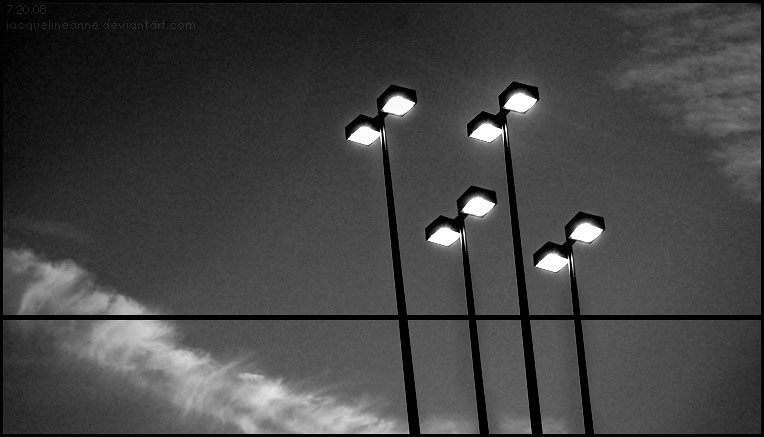This is a detailed black-and-white photograph taken at night, capturing a view looking upward from the ground towards the sky. The image predominantly features four parking lot lamp posts, positioned slightly to the right of center. These lamp posts include two that are tall and two that are slightly shorter, all projecting upwards to about the middle of the frame. Each post culminates in a T-shaped fixture with square lamp heads that direct light straight down, and they are clustered closely together, indicating they are part of a group illumination setup rather than street lighting.

A noticeable feature is a black, horizontal line traversing about one-third of the way up from the bottom of the photograph, which could be a physical element like a power line or an artifact from the image capture. The sky in the background is mostly clear except for some cloud formations: one stretches from the left side of the frame towards the center, and a smaller cloud is visible in the upper right corner. Additionally, there is a diagonal condensation trail from an aircraft originating near the center bottom and extending to the left. The street lamps are illuminated, and the overall focus of the image is sharp and clear, emphasizing the contrast and details of the scene.